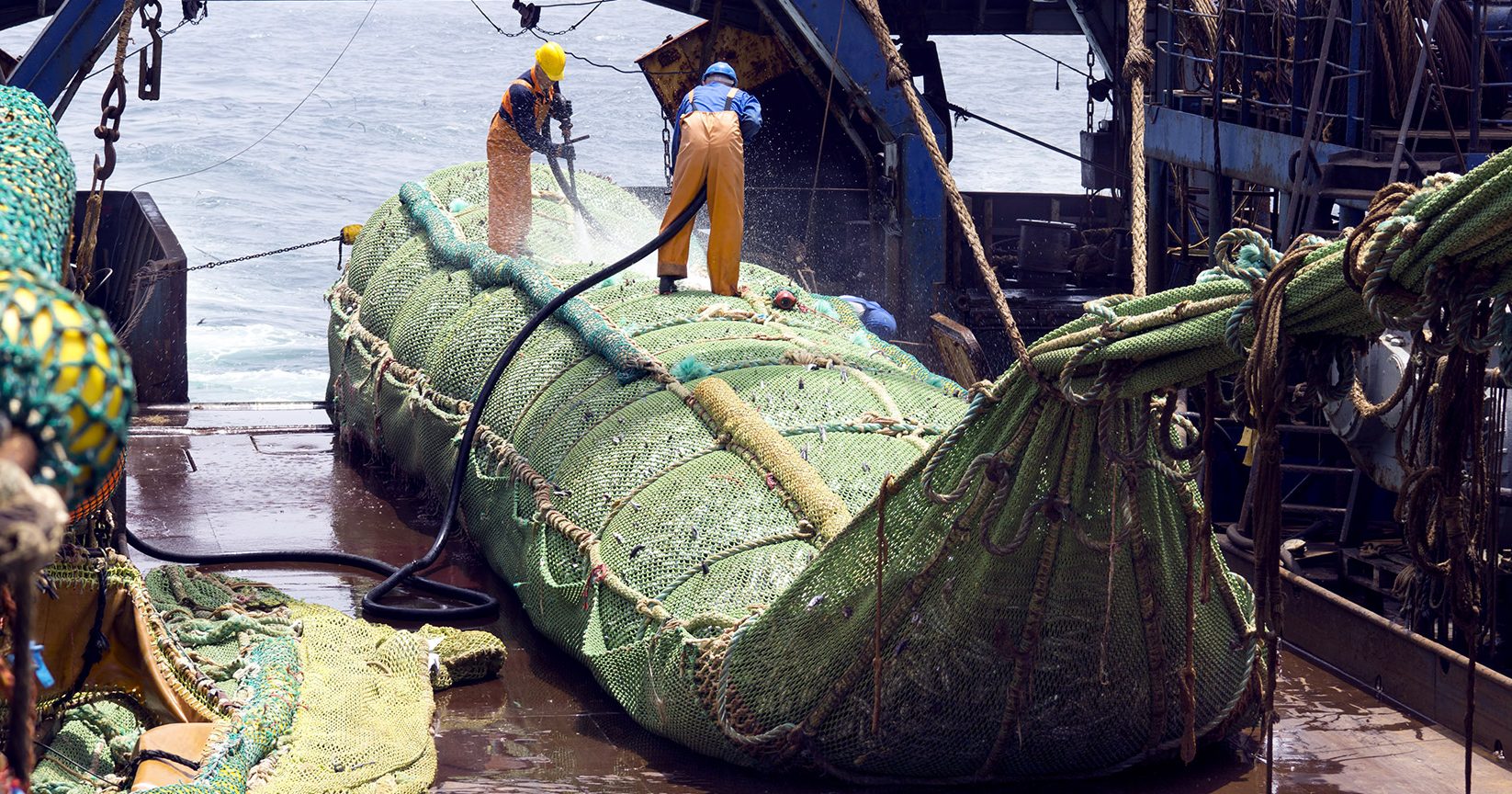In this image, we see a large fishing vessel with a brown deck, cluttered with rigging and equipment. On the deck, two men are standing atop a massive green net filled with what appears to be a large haul of small, indistinguishable fish. The men, both clad in orange rain suits and hard hats—one with a yellow helmet, the other with a blue helmet—are busy spraying down the net with hoses, ensuring the wet deck remains slippery and shining under the equipment-laden scaffolding. The deck is strewn with large brown ropes and blue metallic structures, supporting additional netting and tangled rigging on both the right and left sides of the ship.